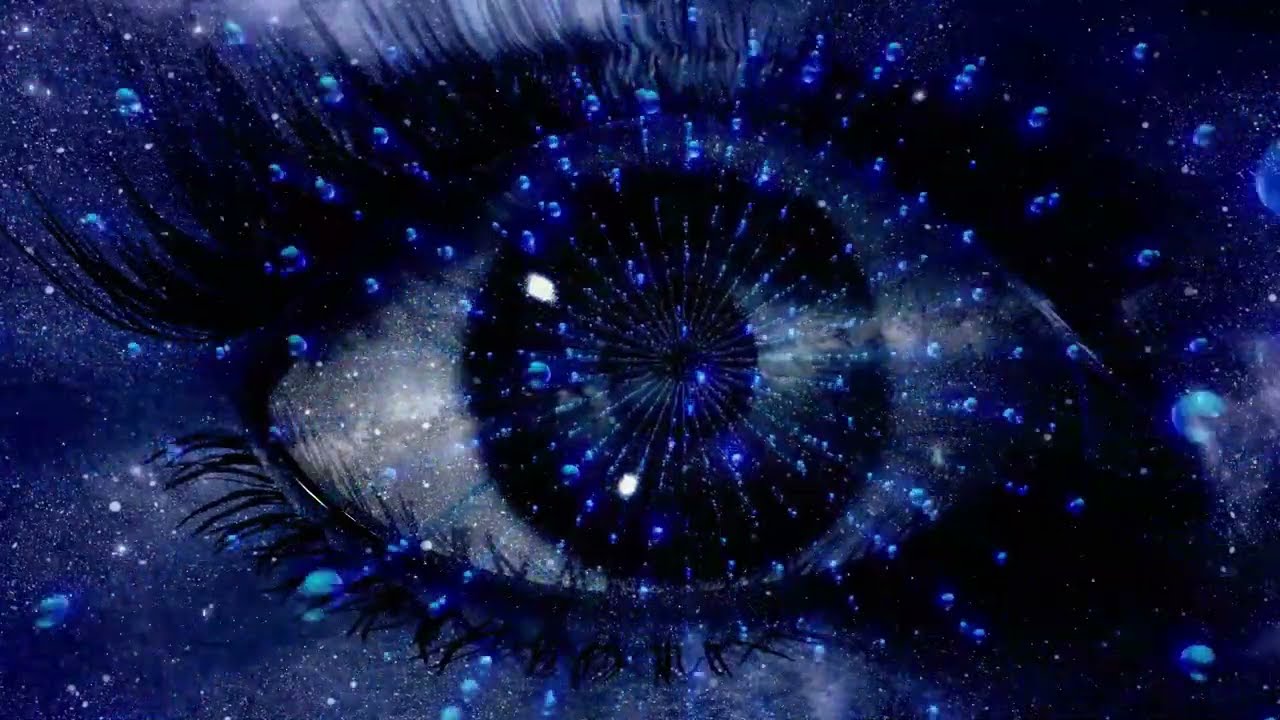This image is a stylized, close-up artistic rendition of a human right eye set against a cosmic night sky. The eye, opened wide to reveal the white sclera above and below the iris, is the focal point in an environment rich with stars and celestial objects. The entire scene is rendered in deep blue and black hues, punctuated by white specks that resemble stars. Long, heavy eyelashes, as if coated with mascara, frame the eye and add a dramatic effect. From the pupil, rays composed of what appear to be celestial objects and blue spheres shoot out radially, creating the impression of a cosmic burst emanating from the eye. This intricate and detailed portrayal combines elements of human anatomy with the vastness of outer space, creating a mesmerizing and surreal image.